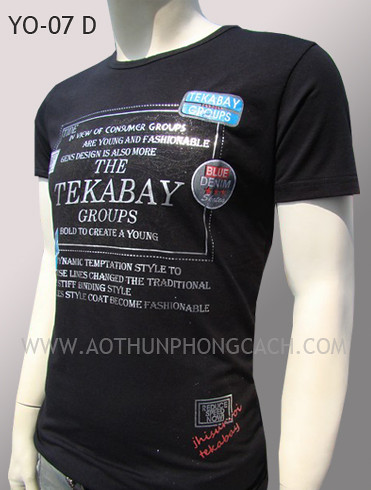The image features a detailed display of a black t-shirt on a white mannequin against a plain grey or white background. The t-shirt is heavily adorned with text, with the most prominent line reading, "Tika Bay groups." Beneath this main text, additional lines mention "Kormor groups" and "young and fashionable Jen's design," although some parts are less clear due to the poor resolution. The shirt also features a distinctive white border around the text, accented by a dotted pattern. In the top left corner of the image, there is a watermark that reads "YO-07D." At the bottom, the website "www.aothunphongcach.com" is visible. The overall style and numerous text elements on the t-shirt suggest it is a trendy, youth-oriented design, possibly aiming to promote fashionable lifestyle themes.